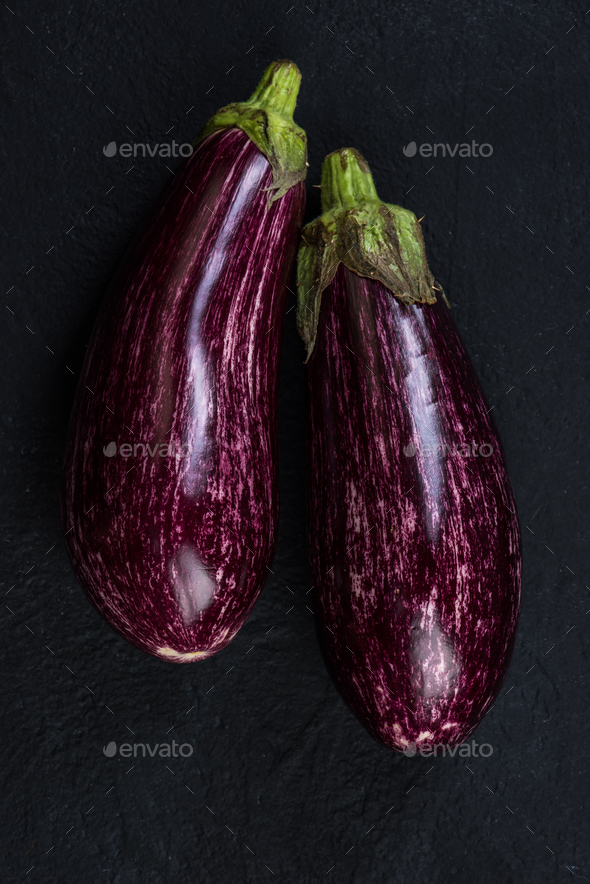The photograph features two eggplants resting side-by-side on a black, possibly textured surface, creating a striking contrast. The eggplant on the left is slightly higher than the one on the right by about two inches. Both eggplants exhibit a rich purple hue interspersed with lighter, almost white streaks throughout their bodies. Each eggplant retains its green, somewhat dirty leaves at the top, with the leaves of the right eggplant cascading further down. The fruits appear to have been picked a while ago, as suggested by the condition of the leaves. The image is overlaid with a semi-transparent gray watermark that reads "Envato," along with a small leaf symbol, repeated six times in a criss-cross dotted line pattern across the photograph.